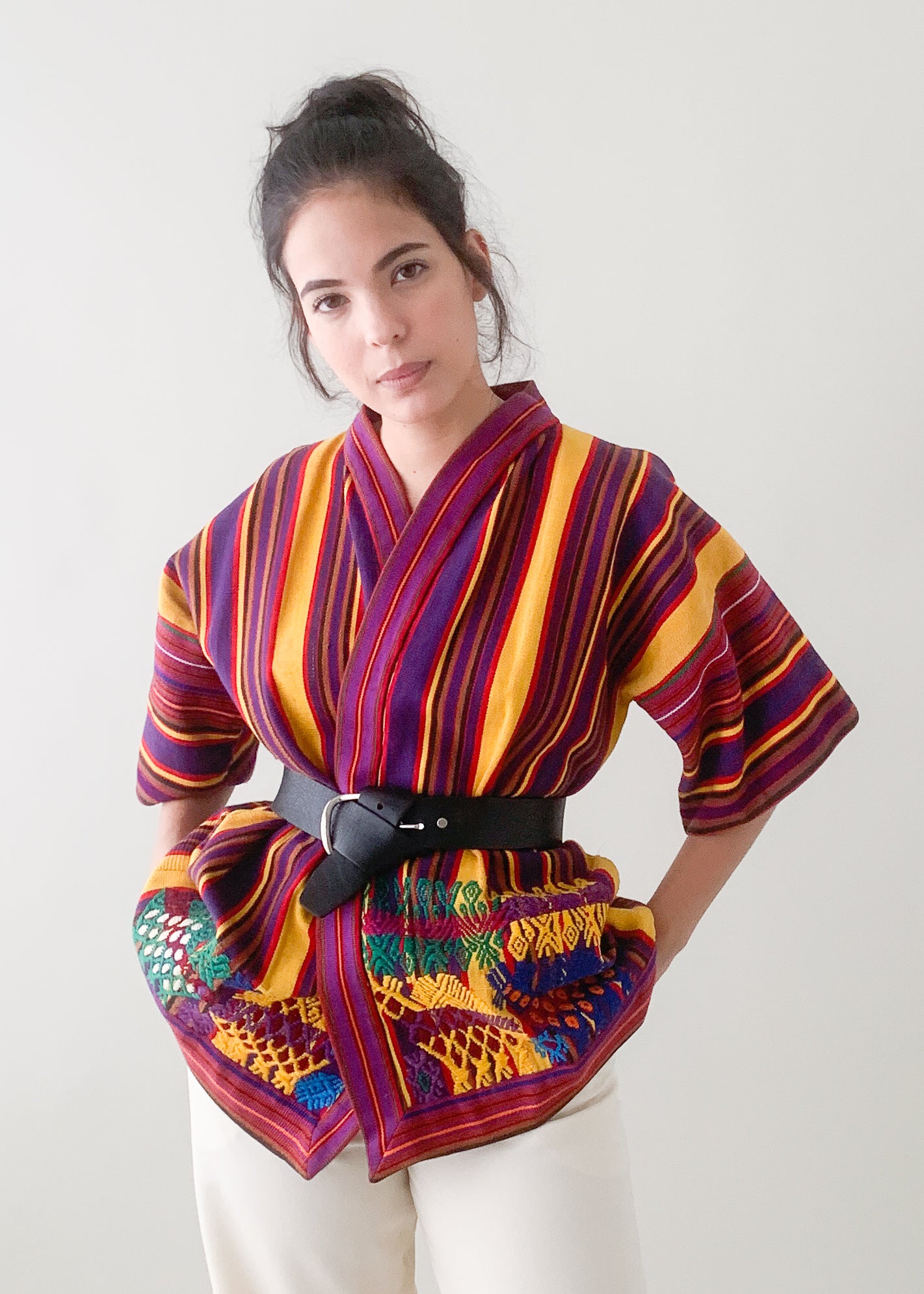In this image, a woman stands against a light gray background, posing slightly tilted to her right while gazing directly at the camera. She has black hair styled in a bun with a few loose strands framing her face. She wears an eye-catching, kimono-inspired tunic that features vivid vertical stripes in hues of purple, yellow, pink, and red. The tunic is short, resembling a shirt with loose sleeves that reach her elbows. It is cinched at the waist with a black belt, keeping it securely closed. The bottom of the tunic showcases intricate embroidery with yellow, blue, green, and gold crochet patterns. Paired with the tunic, she sports off-white slack pants, with her hands casually tucked into the pockets. Her expression is neutral with a faint smirk, adding an air of subtle confidence to her pose.